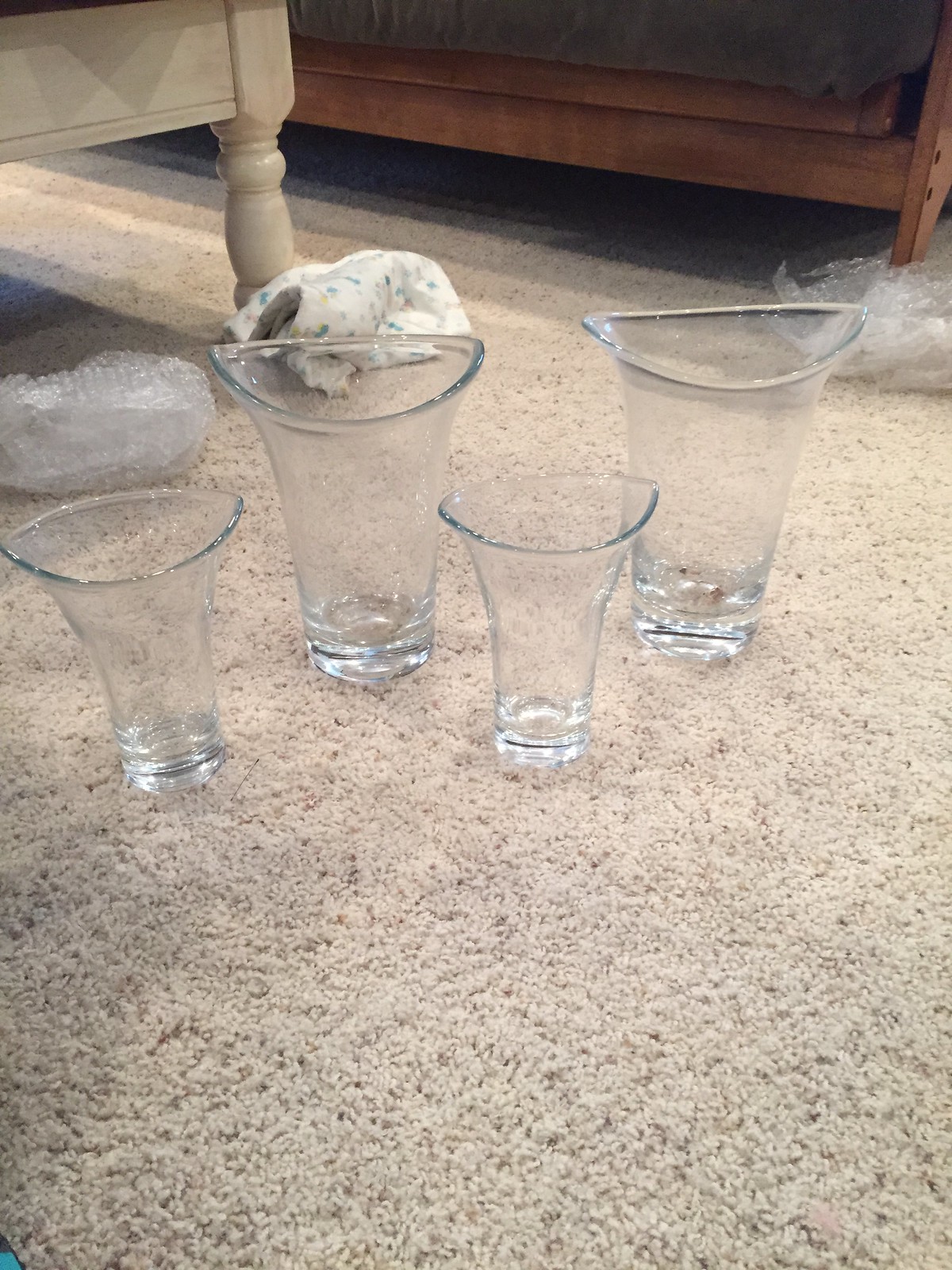In the image, there are four uniquely shaped glass cups, arranged in a sequence from big to small, all sitting upright on a beige carpeted floor. The two larger cups are identical, as are the two smaller ones, and their design features a semi-circle base that flattens out, making them ideal to be placed against a wall or other flat surfaces. This innovative design highlights their practicality. Surrounding the cups are signs of recent unboxing, including bubble wrap and some paper packaging materials scattered on the floor. The setting appears to be a cozy living room, as evidenced by the nearby couch and coffee table, along with additional background elements like bags, more bubble wrap, and what seems to be a white dresser near a bed or another couch.